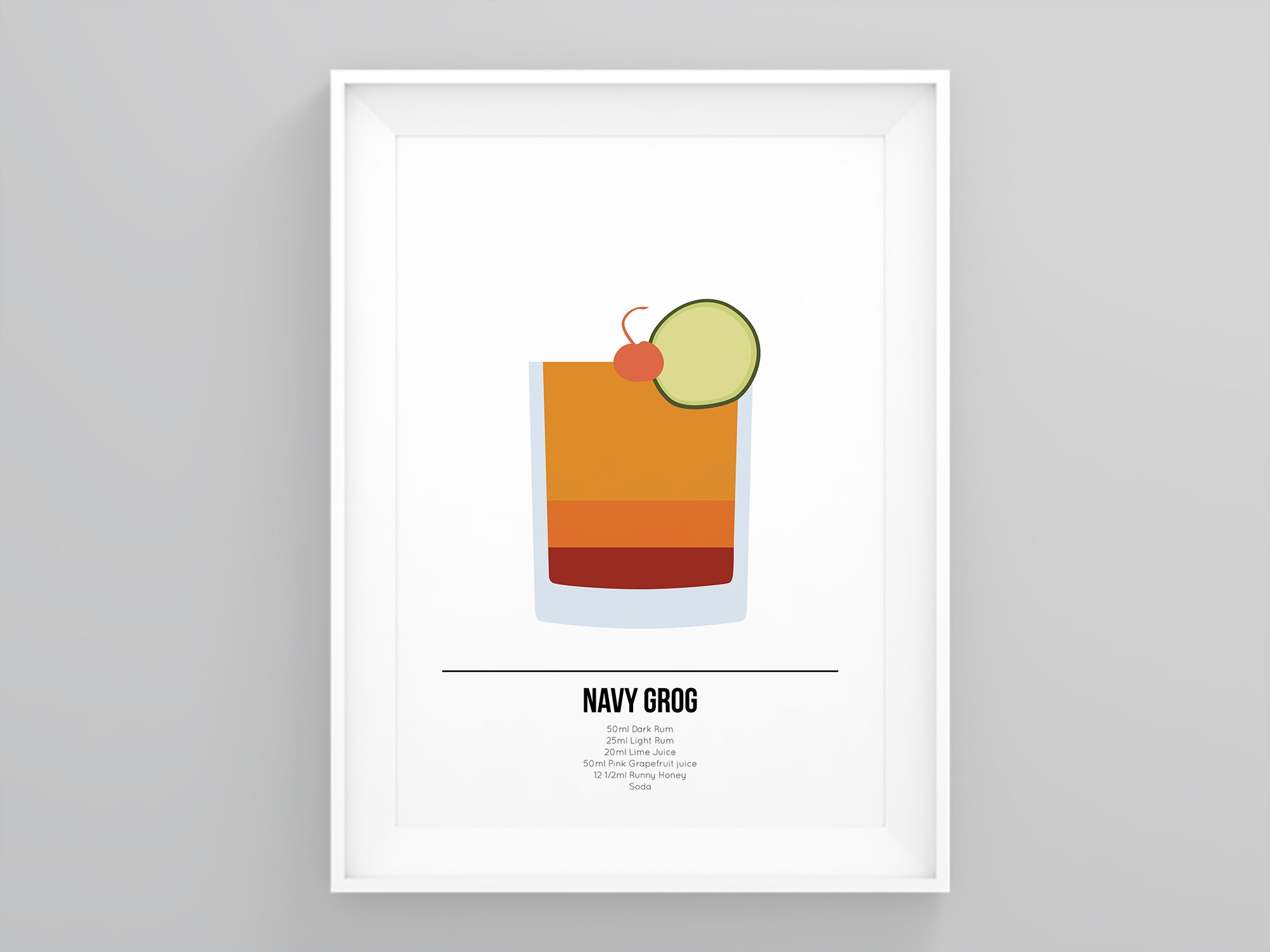This detailed caption is of a framed artwork depicting the Navy Grog cocktail. The image is set against a light gray background, enclosed in a white rectangular frame that measures approximately six inches wide by five inches high. Notably, the left and right edges of the gray backdrop appear slightly brighter than the top and bottom. 

Within this frame lies a smaller, centered illustration that is roughly two inches wide by three inches high. This inner picture features a stylized depiction of a clear glass outlined in a very light bluish gray. The glass is filled with three distinct bands of color: a lighter orange at the top occupying the upper half, followed by a dark orange, and finally a reddish-brown band at the bottom. Atop the glass sits a cherry alongside a lime slice. 

Below the glass is a horizontal black pinstripe that stretches from left to right, acting as a divider between the illustration and the text beneath it. The caption "Navy Grog" is displayed in large black print, and underneath that, the recipe for the cocktail is listed in smaller, lighter print. The recipe reads: 50 milliliters dark rum, 25 milliliters light rum, 20 milliliters of lime juice, 50 milliliters pink grapefruit juice, 12.5 milliliters of runny honey, and soda.

This artwork, portraying a classic mixed drink, might be part of a menu or simply a decorative piece on a gray wall.